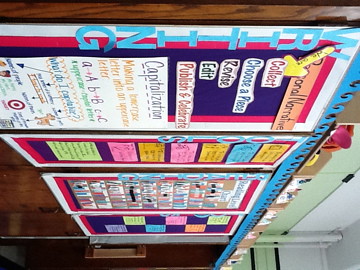The image depicts a classroom wall turned sideways, featuring a multi-colored bulletin board adorned with numerous educational posters and writing samples related to English grammar and spelling. The wall transitions from white to olive green and has black stripes near the top. The board is built with blue construction paper and bordered in layers of white, purple, and blue. It displays headings such as "Capitalization" and processes like "personal narrative," including steps: collect, choose a piece, revise, edit, publish, and celebrate. There are examples showing how to transform lowercase letters (like "a" and "v") into uppercase, all in an array of vivid colors including red, blue, purple, green, orange, and light blue. In the right-hand corner of the image stands a support beam painted in olive green and white, while dark brown wooden doors align the room and a white ceiling hovers above.